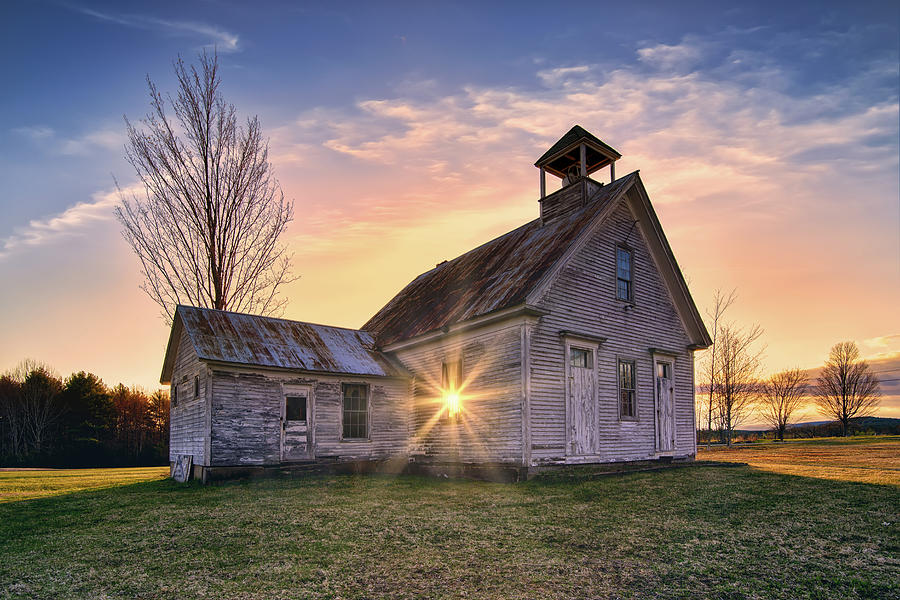This captivating photograph depicts an old, weathered farmhouse or possibly a schoolhouse, framed beautifully against a vibrant backdrop of a sunrise or sunset. The sky is adorned with a gradient of rich blues at the top, transitioning into delicate pinks, warm oranges, and luminous yellows as it meets the horizon. Below this picturesque sky lies a lush expanse of green land, with a patch of flat grass enveloping the building. The house is constructed of whitewashed, wooden slats that have aged and weathered over time, revealing a rustic charm.

The main structure is a single-story building with an attic window on the front, suggesting the possibility of a second floor. The front facade features two large doors that are white but heavily weathered and appear to be boarded over. Between these doors is a single window. On the right side of the building, an additional structure extends out, seemingly built later, and includes another door and a window, both similarly weathered.

A notable feature of the building is the bell tower perched on the roof, hinting at its potential history as a church or a schoolhouse. The roof itself is black, tinged with rust, further emphasizing the building's age and exposure to the elements. Adding to the scene's allure, a beam of sunlight pierces through the left window of the side extension, casting a radiant starburst of light. 

The surrounding landscape is dotted with trees, some evergreen and some barren, suggesting the season might be late autumn or winter. A particularly tall, leafless tree stands immediately behind the house, accompanied by a grouping of other bare trees and a forest in the distant background. The absence of a driveway or visible pathway enhances the feeling of isolation and timelessness, making this scene reminiscent of a moment frozen in history.